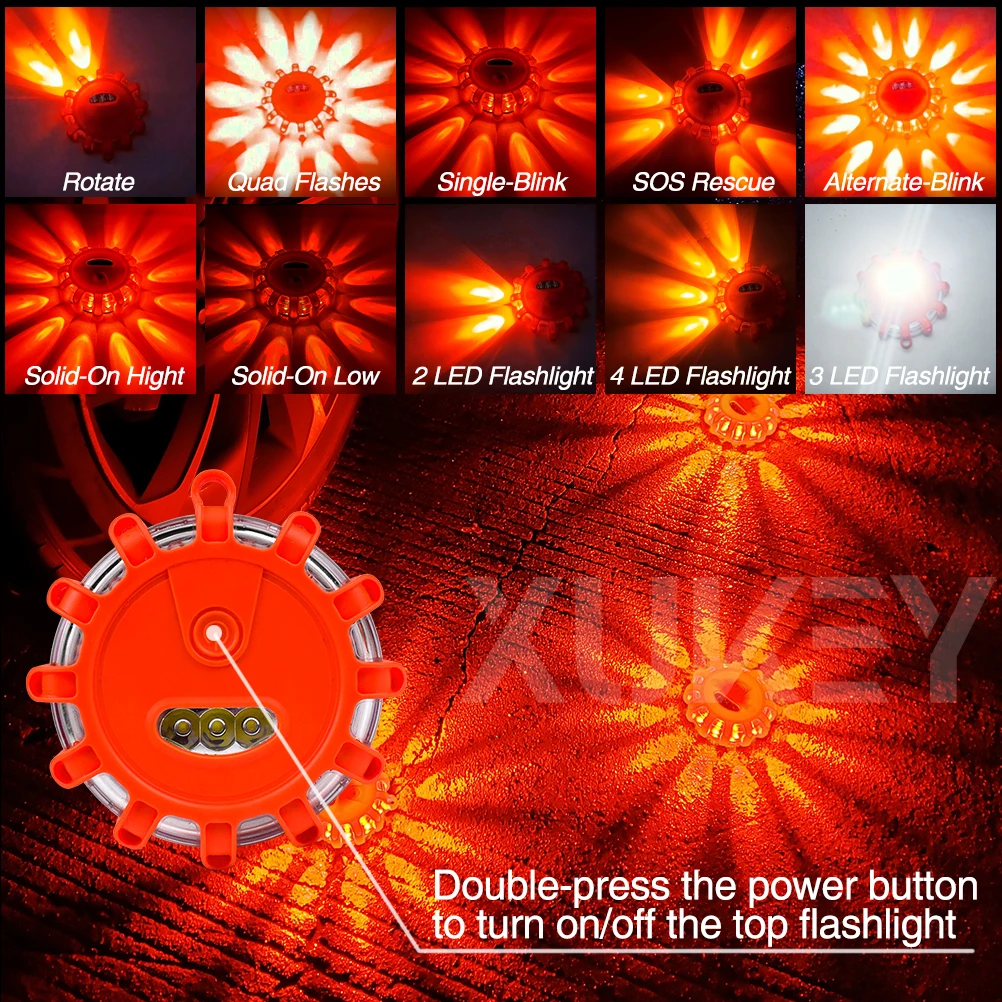The vividly red poster prominently features a detailed advertisement for the multi-functional XU-Key flashlight. The main colors of the image are strikingly orange, red, and black. A close-up in the lower right-hand corner highlights a circular component with batteries, accompanied by a directive in white text: "Double press the power button to turn on/off the top flashlight." Above this, the top two-thirds of the poster is organized into ten smaller panel photos arranged in two rows, each depicting a different mode of the flashlight. From left to right, they are labeled: Rotate, Quad Flashes, Single Blink, SOS Rescue, Automatic Blink, Solid on High, Solid on Low, 2 LED Flashlight, 4 LED Flashlight, and 3 LED Flashlight. Most of these panels demonstrate vivid red, orange, and black light patterns, except for the 3 LED Flashlight in the bottom row on the extreme right, which shows a clean, solid white light.